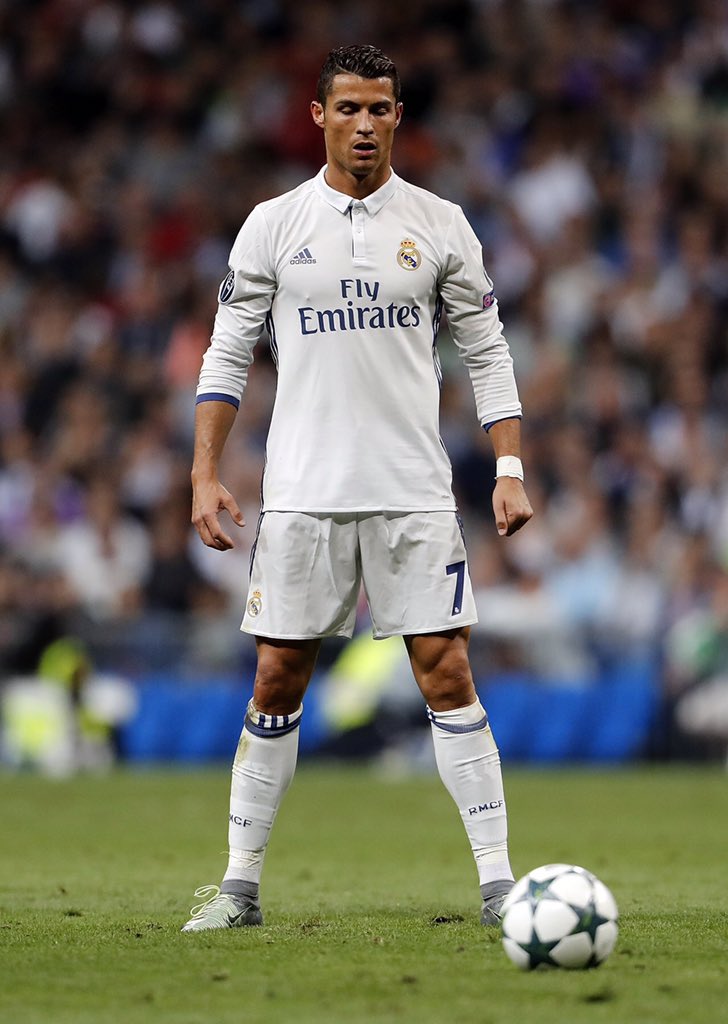The image captures Cristiano Ronaldo, a dark-skinned soccer player with dark hair, standing on a green soccer field. He wears a white long-sleeved jersey with "Fly Emirates" emblazoned on it, white shorts marked with the number 7 in blue, and complete white gear including wristbands, socks, and shoes. Ronaldo stands with his arms by his side and legs apart, eyes cast down towards a white soccer ball adorned with green stars at his feet. The background showcases a blurred stadium filled with indistinct fans, emphasizing the sharp focus on Ronaldo as the central figure.